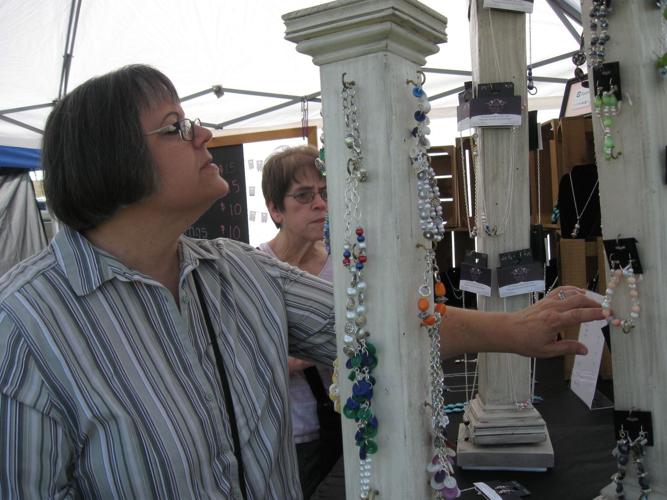In this detailed outdoor photograph taken at a bustling festival or flea market, two elderly women are intently browsing a jewelry stand under a white tent. The centerpiece of their interest is a peach-colored bracelet, which one woman, sporting short gray hair, bangs, and oval glasses, holds delicately in her left hand while clad in a light green striped button-up shirt. Displayed on white pillar mounts beside her, an array of homemade jewelry—including bangle bracelets, necklaces, and earrings in vibrant hues of silver, blue, green, orange, and purple—captures their attention. Behind her, another elderly woman with short, balding hair and glasses peruses the stand's offerings, including pieces priced at $15, $5, and $10 as indicated on a see-through glass panel. The scene is set against a cloudy sky, with pastel colors and wooden storage objects in the background, enhancing the charm of this lively market day.